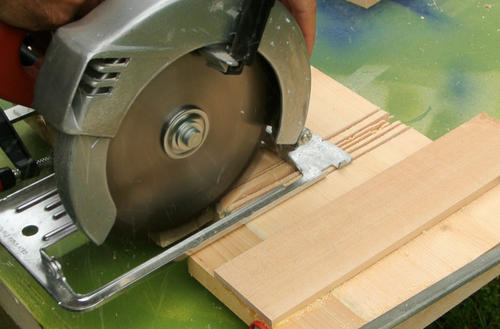The image depicts a top-down view of a home project in progress, centered around the use of a table saw and a circular saw. The work surface is a greenish-blue formica countertop, supporting several pieces of light tan to light brown wood with darker grain patterns. Some of the wood has already been cut, showing marks from previous cuts, while other pieces are positioned to be sawn. 

A circular saw, with visible metallic safety guards and a dark gray stainless steel blade housing, is actively in use, guided by a person's hand just visible holding the blade guard. The circular saw is slightly outdated but functional, cutting a notch into the wood through multiple passes. The scene emphasizes the precision and care involved in the project, illuminated by the light wooden hue against the colorful background, all devoid of any writing or additional elements.